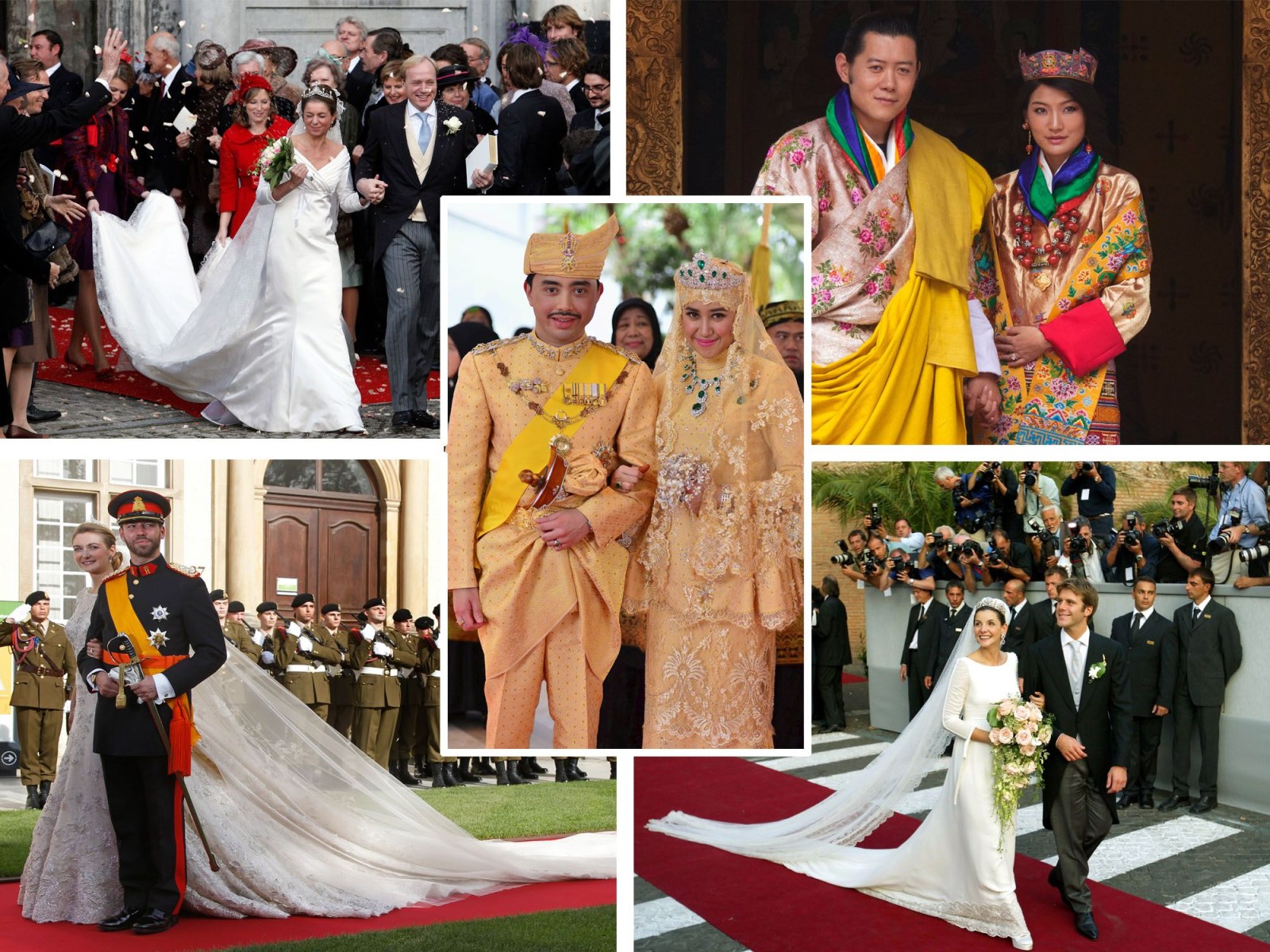This is a meticulously crafted collage of five wedding scenes from various cultures, each depicted in rich detail. The central image features a couple in peach-yellow traditional garments; the groom dons a yellow sash and hat, while the bride is dressed in a long-sleeved shirt and skirt with white lace, completed by a jeweled headdress. Surrounding this central image are four distinct scenes:

- The top left corner shows a bride in a white wedding dress with a red-clad attendant carrying her train, walking on a red carpet outside a grey building, likely part of the English royal family, accompanied by dignitaries in black and grey suits with blue ties.
- The top right depicts an Asian couple in matching multicolored robes adorned with floral patterns, holding hands against a dark background.
- The bottom left features a bride in a white or pinkish gown standing next to a groom in a dark uniform with a sword and silver badges, his uniform possibly dark blue or green with a red-striped hat.
- The bottom right captures a classic American wedding scene, with the bride in a white dress holding a bouquet and the groom in a traditional black tuxedo. They walk on a red carpet flanked by guests in dark suits and white shirts.

The entire collage bursts with colors, including black, white, grey, red, yellow, peach, green, orange, some purple, and brown, beautifully showcasing the diversity and splendor of wedding traditions from around the world.